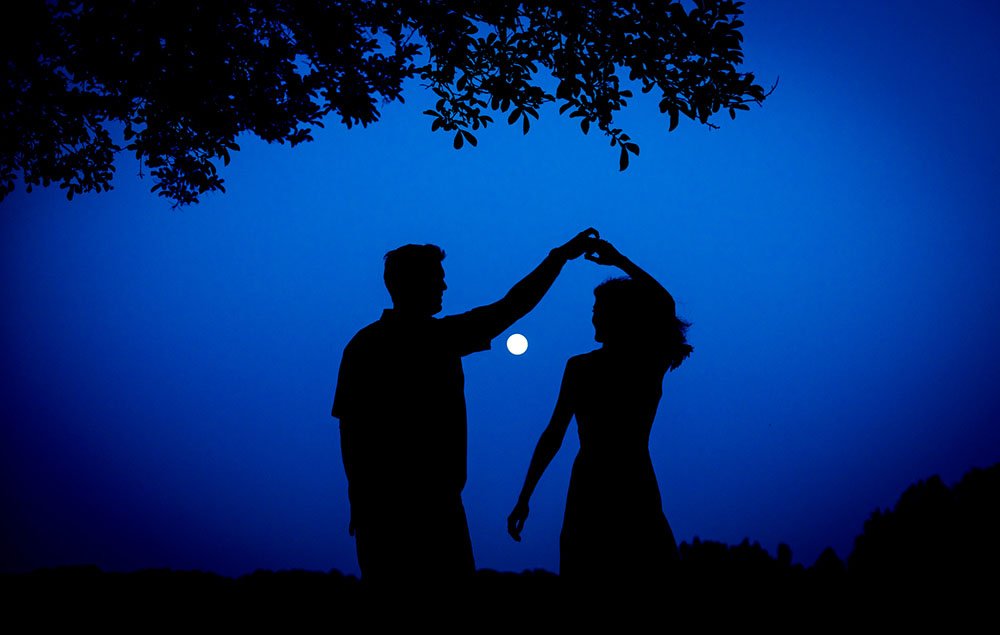In this digital nighttime photograph, a man and woman stand as black silhouettes against a strikingly deep blue sky that brightens slightly toward the center. They are holding hands above her head, with the man's left hand connecting to the woman's right. The woman, seemingly dressed in a flowing dress, faces the man while walking towards a small, radiant white moon that sits almost centrally in the image. The man, appearing to wear a short-sleeved collared shirt and pants, is facing her. Her hair cascades past her shoulders. The top left of the image features the black silhouette of a tree canopy casting over them, while the bottom right shows a varied treeline of indistinguishable bushes and shrubs, all cloaked in darkness. The moon is perfectly framed by their uplifted arms, making for a mesmerizing and intimate scene.